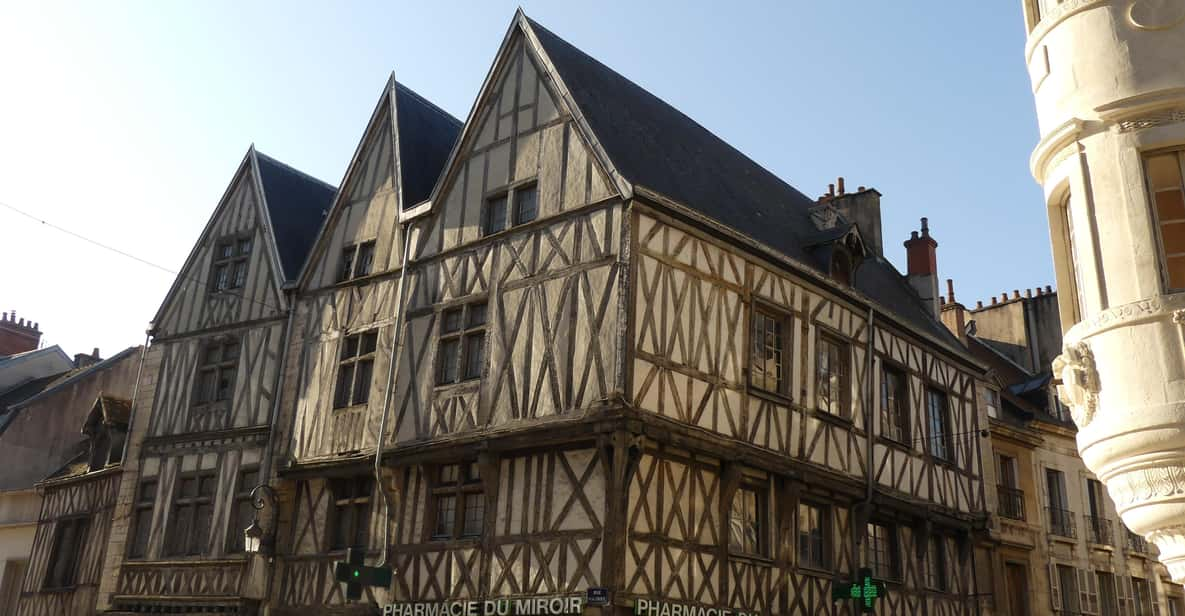This photograph captures a quaint corner building set against a clear blue daytime sky with light streaming in from the upper left. The building, approximately three stories tall, is predominantly light brown with dark wood accents arranged in a cross pattern within the rectangular panels adorning its facade. The structure, evocative of European architecture from the 18th or 19th century, integrates modern elements such as neon signage and lighting. A notable feature is the twin-pointed roof and several chimneys that crown the building. Signage on the two visible corners reads "Pharmacie du Miroir," suggesting it functions as a pharmacy. This blend of historical architecture and current-day modifications suggests an old-timey setting revitalized for contemporary use.